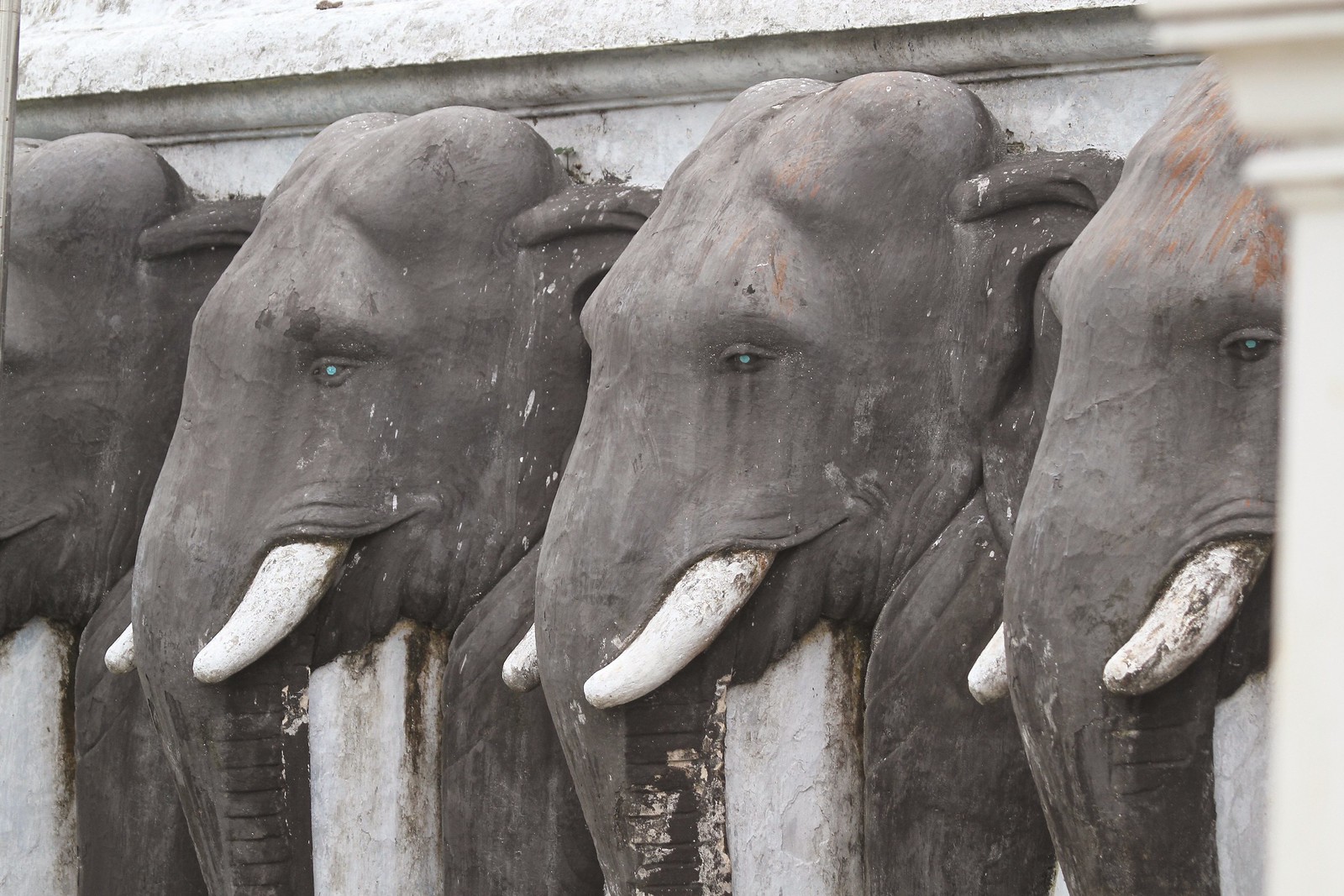This photograph showcases a detailed sculpture of four elephant heads, carved intricately out of a distressed stone wall that exhibits a mix of white, gray, and brown hues. The wall features a rounded upper border that flattens out into the sides. Each elephant head seems to emerge from the wall, giving a three-dimensional effect. Their skin is painted a realistic dark gray, with hints of reddish-brown distressing on the tops where the paint has weathered. The elephants sport large, flappy ears and long, downward trunks ending near their feet. Their tusks are ivory white, contrasting with their aqua green eyes that hold a touch of baby blue, although the eyes of the elephants are described slightly differently by some sources. A white pillar is visible in the right corner of the photo, adding to the architectural detail of the stone wall. The composition includes all four elephants, though the one on the far left is partially out of focus and cut off by the photo's border. The elephants appear to be approximately the same size but show varying degrees of wear and detail, adding to the artwork's aged and textured look.